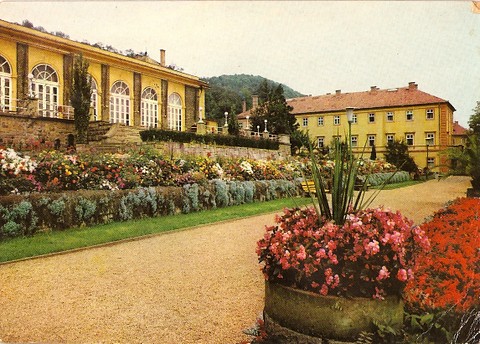This appears to be a scene from an aged photograph, possibly an old Spanish-style image or even a finely executed painting. The image showcases an outdoor setting with two prominent yellow buildings that embody old-world charm, emphasized by clay terracotta roof tiles. On the left, there is a large mansion-like house with expansive, arched, floor-to-ceiling windows, featuring six segments of archways with rectangular glass doors. These segments are adorned with meticulous landscaping of leveled gardens that ascend along a brick wall, adorned with diverse flowers and hanging plants.

To the right, another taller yellow building with multiple floors can be seen. This building features numerous small windows, suggesting it might be an apartment complex or a similar structure. A staircase from the left-hand mansion leads up towards this second structure. Between these elements is a carefully manicured strip of grass, bordered by a pebble pathway. Adjacent to the path on the bottom right is a large, round, stone flower pot, housing a striking arrangement of pink begonias and spiky, dracaena-like stems in the center. 

A large stone wall defines the garden area that sits above, complemented by a smooth stone driveway and pathway lined with colorful flowers and a bench. In the background, rolling hills with trees gently rise, and the white sky suggests an early morning ambiance. The image's aged appearance, with signs of peeling and folding, adds a layer of nostalgia to this vibrant outdoor scene.